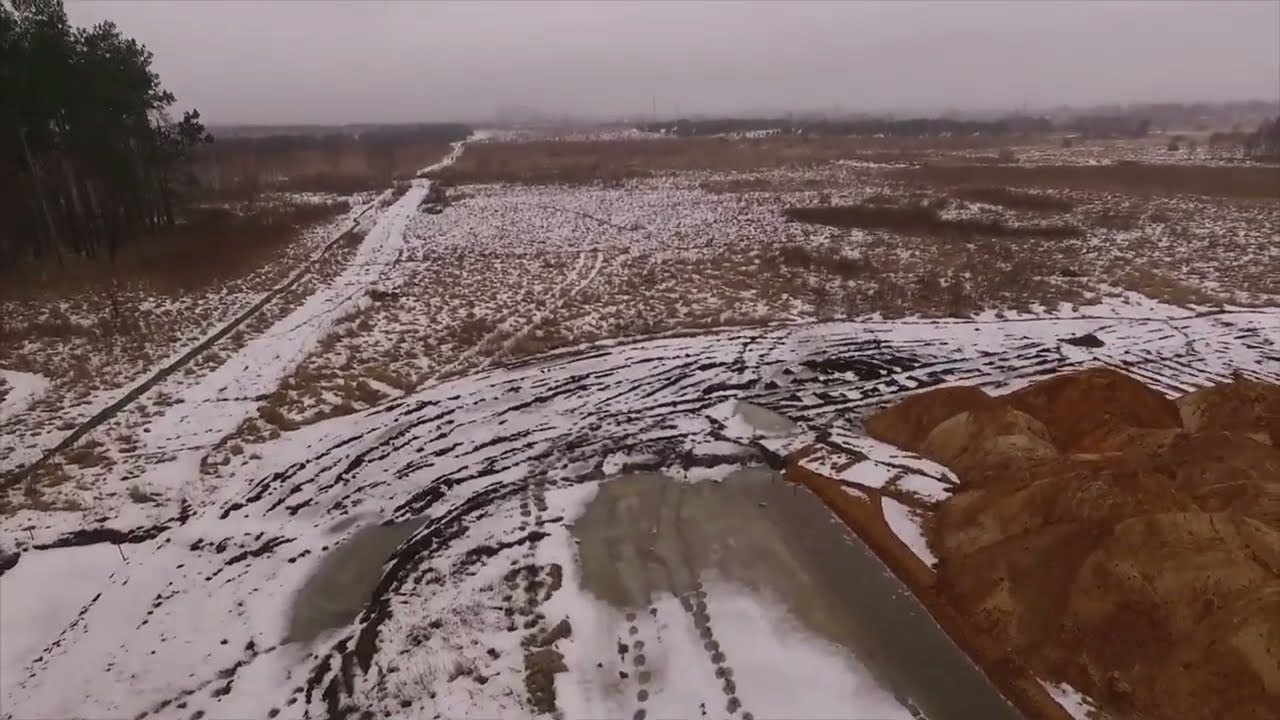In this colored photograph taken outdoors during the daytime in winter, the scene is marked by an overcast, gray sky that lends a somber tone to the image. The ground is mostly covered by a thin layer of snow, rendering it a low-lying, flat area with sparse brown vegetation peeking through, indicating the dead of winter. Two pathways crisscross the snowy terrain: one stretching straight into the distance, featuring visible footprints, and another veering off to the right, showing both footprints and faint tire tracks. The upper left corner of the photograph is dominated by a small group of tall trees, adding a hint of height to an otherwise flat, snow-blanketed landscape. The ground also exhibits several streaks and indentations, suggesting the movement of multiple vehicles that have left grooves behind, especially noticeable in the lower right where reddish-brown dirt is exposed.